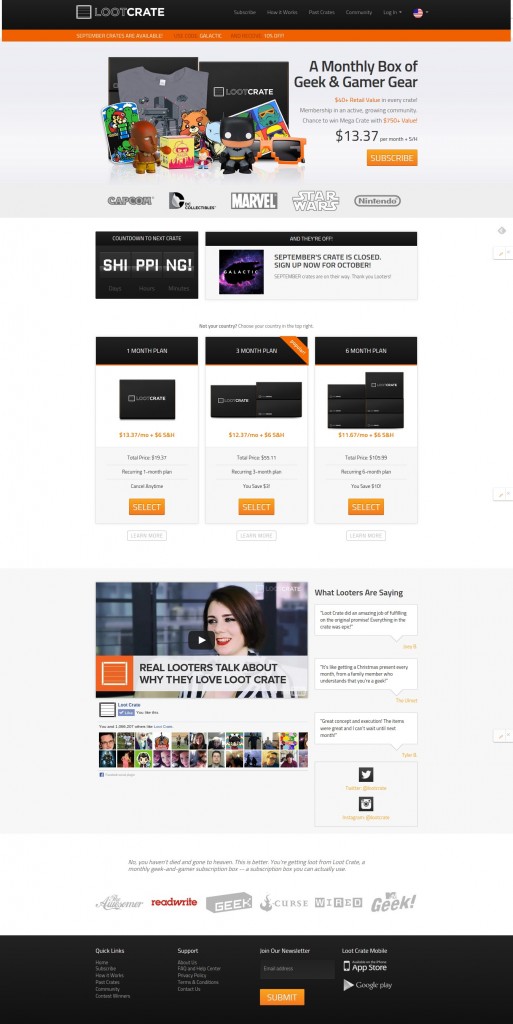This photograph depicts the homepage of a website for Loot Crate, a subscription service catering to fans of geek and gamer culture. At the top of the page, a black header prominently displays the "Loot Crate" logo. Immediately below, an eye-catching orange banner announces that "September crates are available." 

Beneath the banner, a gray section provides a succinct description of the service: "A monthly box of geek and gamer gear." This section visually enhances the message with images of Funko Pops, stickers, and small games, hinting at the type of items included in each crate.

The promotional text highlights the key benefits of the subscription: each box has a retail value exceeding $40, offers membership in an active, growing community, and provides a chance to win a "Mega Crate" valued at over $150. The service is priced at $13.37 per month, plus shipping and handling.

The page lists the brands featured in the crates, such as Capcom, Marvel, Star Wars, and Nintendo, which are sure to attract enthusiasts.

A countdown timer indicates the time remaining until the next crate shipment, fostering a sense of urgency and excitement. Additionally, the site presents various subscription plans: a one-month plan for $13.37, a three-month plan for $12.37 per month, and a six-month plan for $11.67 per month, all exclusive of shipping and handling fees.

At the bottom of the page, testimonials under the heading "What Looters Are Saying" provide social proof of the service's value. A clickable video link titled "Real Looters Talk About Why They Love Loot Crate" offers potential customers genuine insights into the subscription experience.